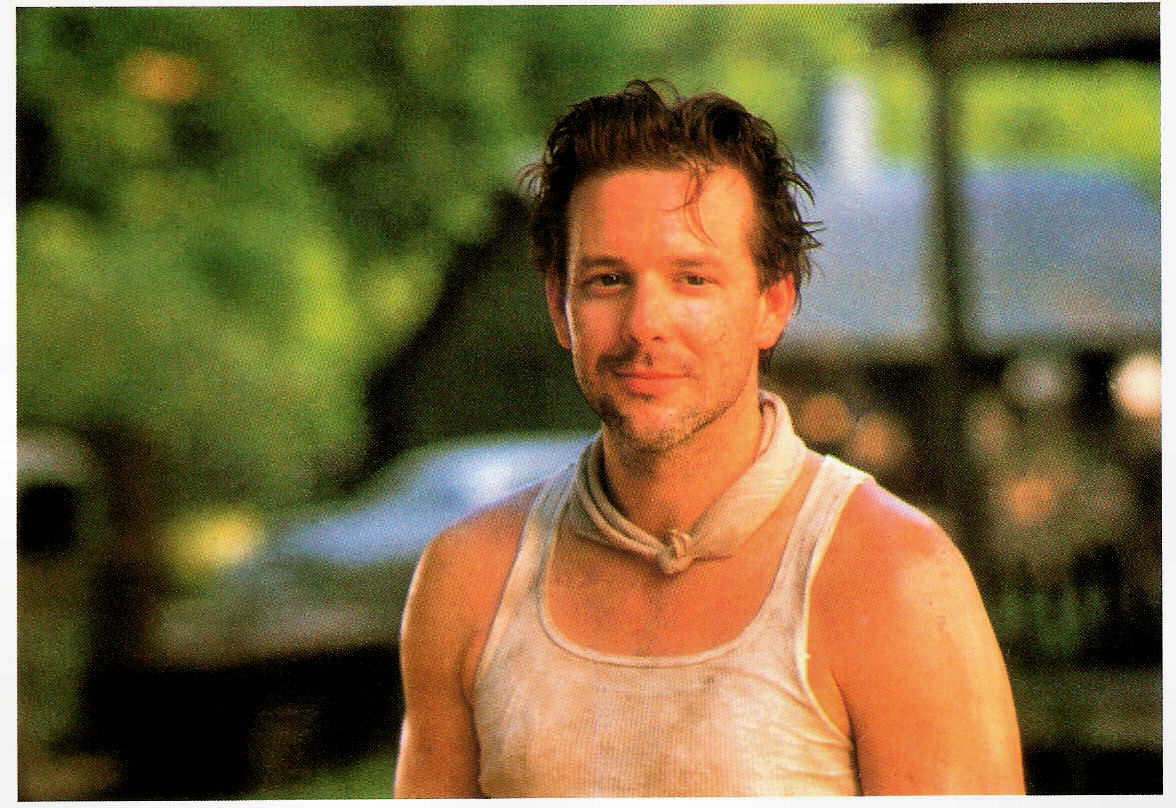The image appears to be a grainy photograph, likely a film still, featuring a young Mickey Rourke. Positioned in the center-right of the frame, Rourke is depicted as a somewhat disheveled character, smiling warmly towards someone off to his right. He wears a dirty, ribbed white tank top, with a white cloth, possibly a neckerchief, tied around his neck. His short, greasy brown hair is characteristically swept back, and he sports a five o'clock shadow, enhancing his rugged appearance. His skin appears sweaty and dust-covered, adding to the gritty feel of the image. The background, though blurry, suggests an outdoor setting with some greenery, possibly trees, on the left and upper parts, and elements like a barn or building structure faintly visible on the top right. A small part of what might be a vehicle can be noticed at the lower left corner, contributing to the scene's rustic backdrop.